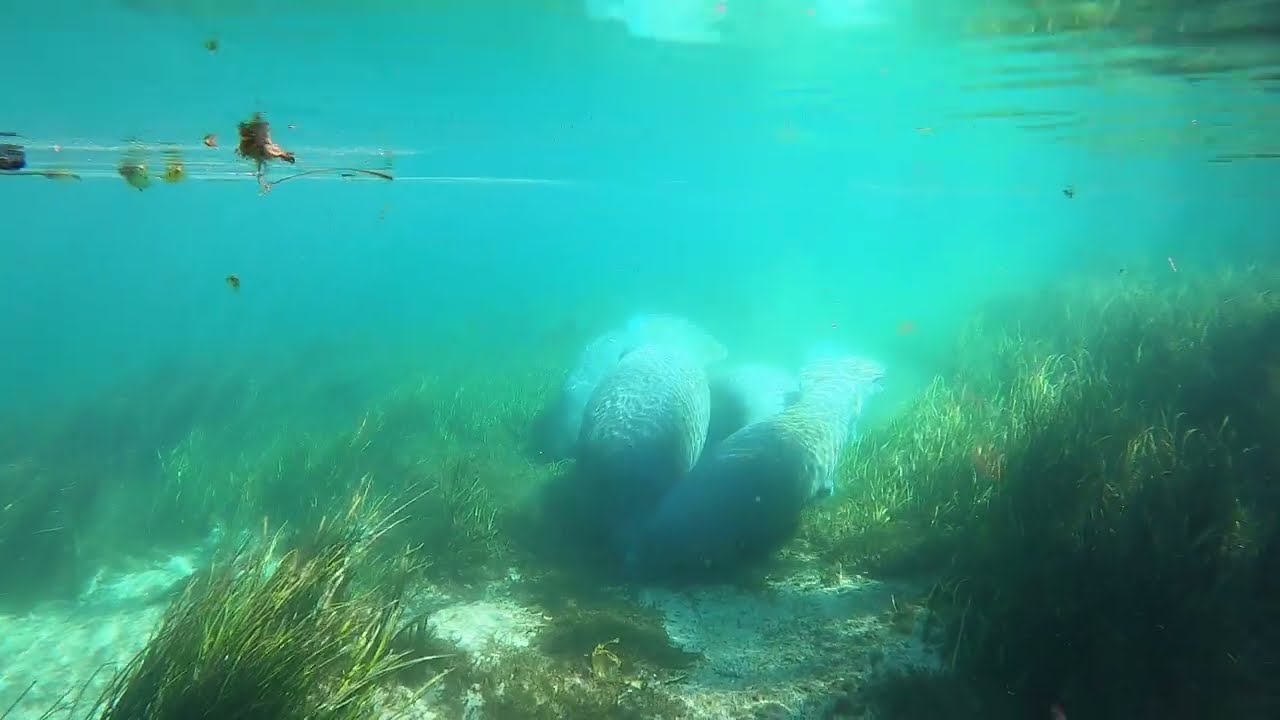This captivating underwater image, taken in a body of water such as a pond or lake, captures the mesmerizing aquatic environment. The water appears turquoise blue but is somewhat murky, adding a mysterious ambiance. The scene is observed from beneath the surface, revealing seagrass or similar long green vegetation growing in the sandy bottom, with more dense patches towards the lower quadrants. Floating atop this vivid underwater scape are leaves and possibly algae, contrasting sharply against the water’s aquamarine hue. Central to the image is a globular structure tinted light gray and greenish-blue. This feature, which might be a smooth rock formation, a plant resembling a cactus with rounded pieces, or a cluster of sea creatures, remains ambiguous due to its blurred appearance. In the upper left, there are ripples and horizontal streaks, suggestive of light penetrating the water surface and debris such as moss or leaves drifting above. This underwater exploration, with its varying shades and indistinct objects, invites a sense of curiosity and wonder.